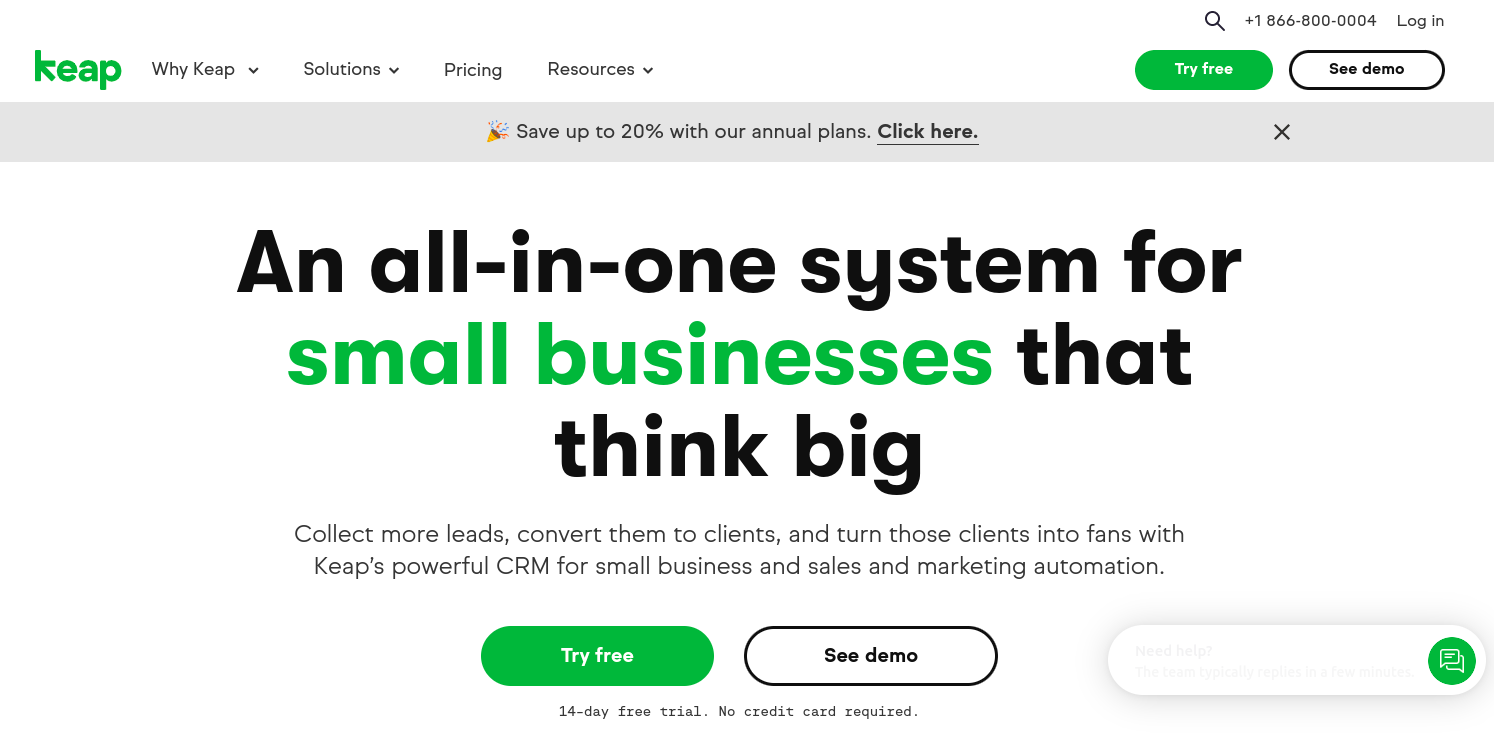**Detailed Caption:**

The screenshot features a user interface with a white background prominently displaying the branding elements and user options for Keap, represented as "KEAP" in green. The top navigation bar includes menu items labeled "Why Keap," "Solutions," "Pricing," and "Resources." Additionally, there is a magnifying glass icon indicating a search function and a customer service phone number displayed as "+1-866-800-0004."

On the right side of the navigation bar, there are options for user login and two interactive buttons: a green oval button with white text that reads "Try Free" and a white oval button labeled "See Demo."

A central message on the page highlights a promotional offer with the text: "Save up to 20% on our annual plans. Click here," with the phrase "Click here" in bold and underlined for emphasis.

Below the promotional message, a green-highlighted statement reads: "An all-in-one system for small businesses that think big. Collect more leads, convert them to clients, and turn those clients into fans with Keap's powerful CRM for small business and sales and marketing automation." This underscores the comprehensive and integrated nature of Keap's services.

Toward the bottom section, there is an additional call to action with another set of interactive buttons: a green oval button with the same "Try Free" text in white and a white oval button labeled "See Demo." nearby, there's an additional white oval featuring a green circle with two overlapping chat bubbles, indicating an accessible chat feature for assistance or queries.

Lastly, highlighted in a distinct section, a notice states: "14-day free trial, no credit card required," ensuring potential users of the ease of trying out Keap’s services without commitment.